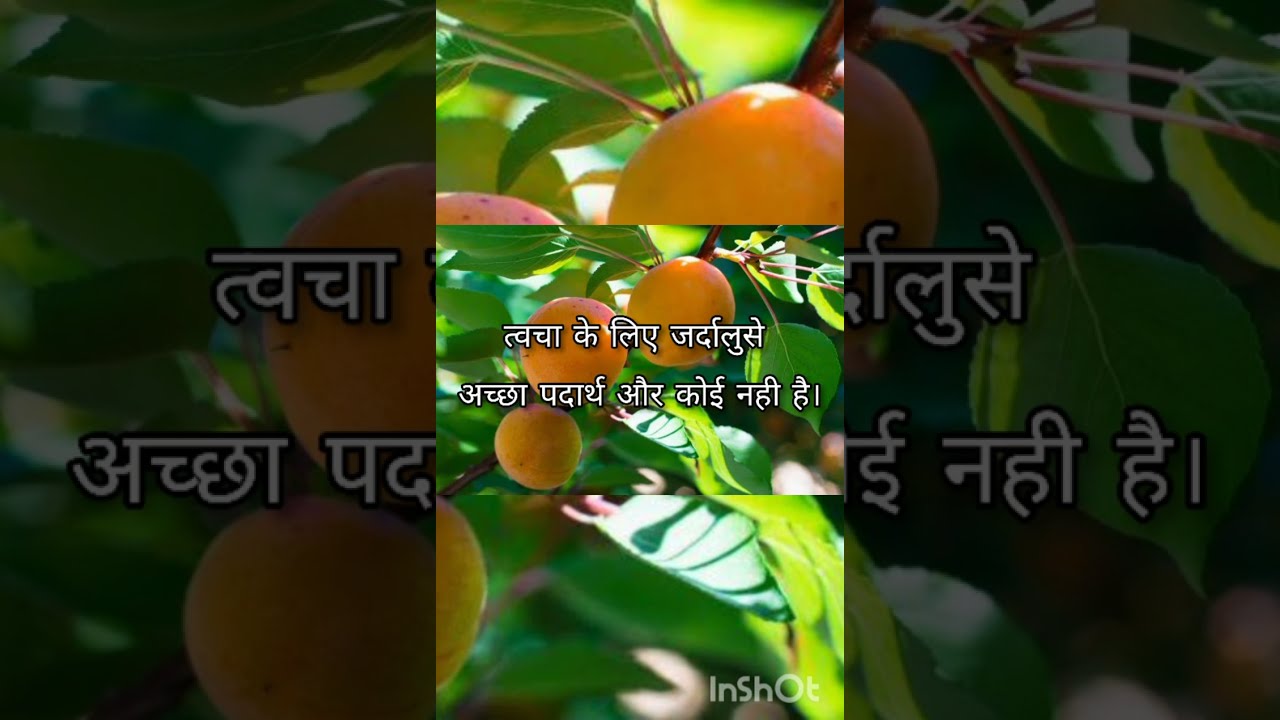In a vertically-taken photograph, likely captured on a smartphone, we see a close-up of a fruit tree bearing three round, orangish-yellow fruits. These fruits, possibly oranges or another type of citrus or Asian fruit, hang amid abundant, vibrant green leaves with visible stems. The fruits appear ripe and exhibit some dot patterns in darker shades. Sunlight filters through the leafy branches in the background, adding to the image’s natural charm. The composition is layered, with the smaller central image overlapping a larger version of itself in the background, creating a visually intriguing effect. Superimposed on the image are white foreign characters in a language unknown to the viewer, and at the bottom, the word “InShot” is visible in faded white lettering.